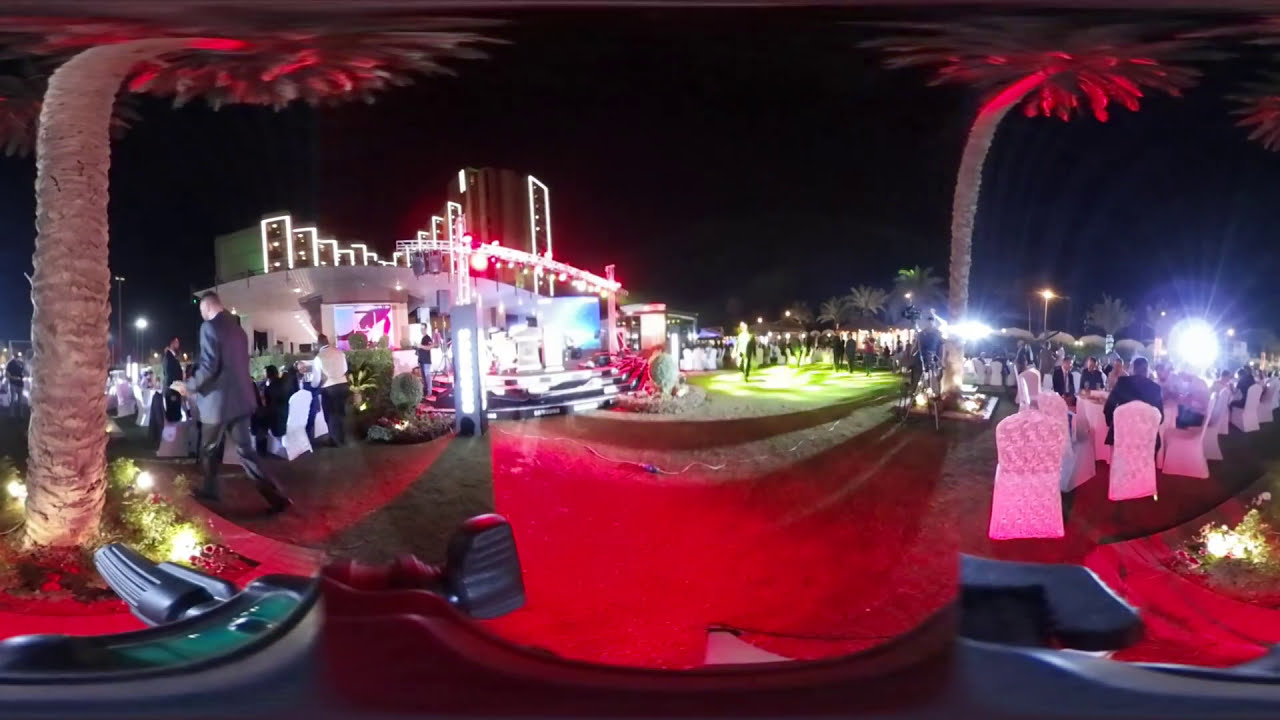In this outdoor nighttime scene, the sky is enveloped in darkness. A prominent palm tree stands on the left side, its crown illuminated in red. More palm trees are scattered around, their tops also glowing with red lights. To the center-left, a well-lit building or possibly a hotel can be seen in the distance. 

The focal point of the image features a brightly lit area, possibly a dance floor or stage, adorned with stage lights and surrounded by people celebrating. This likely festive event, potentially a wedding or concert, sees attendees dressed formally in suits and dresses. There are groups of people sitting and mingling around white-clothed tables and premium-looking white chairs, indicating a formal setup.

On the right side of the image, additional seating is arranged with similar tables and chairs, all under the illumination of spotlights cast from the stage. A red carpet runs through the area, adding to the upscale atmosphere. Overall, the image captures a lively and elegant event, with people joyfully congregating amidst the glow of lights and the serene presence of palm trees.